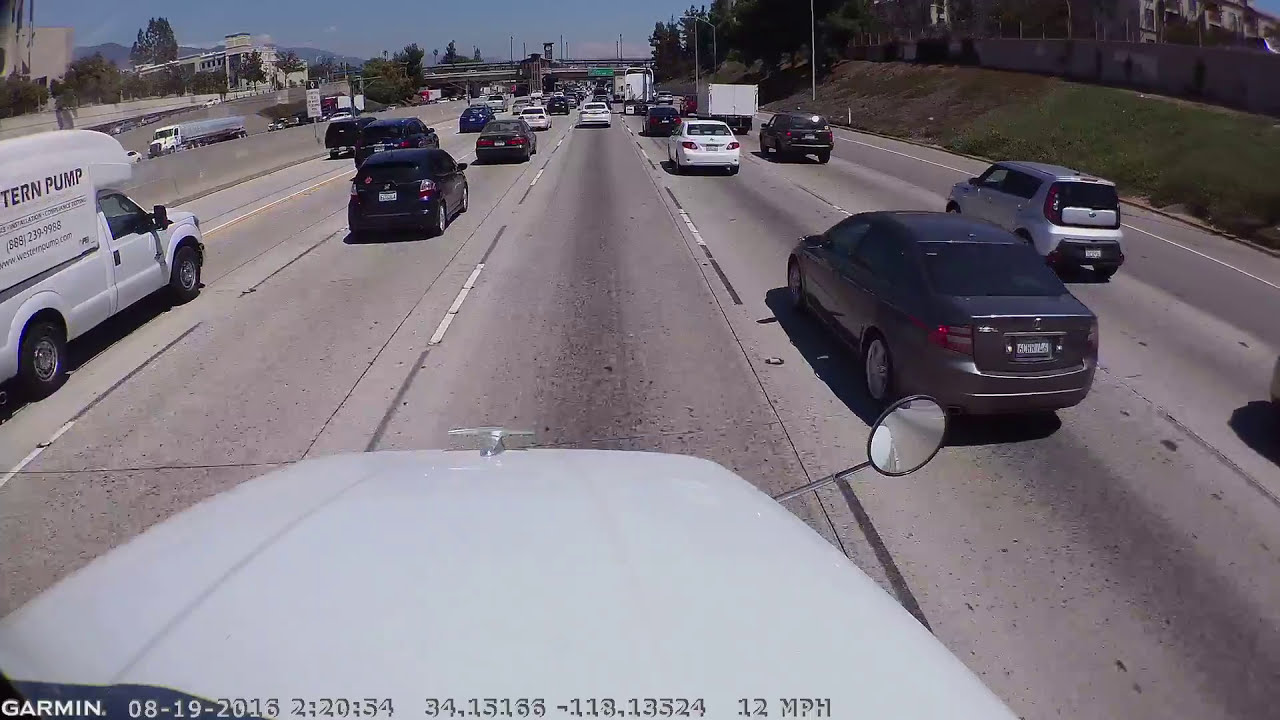This image captures a five-lane expressway bustling with vehicles under a clear blue sky. At the bottom of the picture, a Garmin timestamp reads 08-19-2016 22:20:54, along with coordinates and a speed of 12 miles per hour. The scene is viewed from the vantage point of a large truck, identifiable by its white hood and prominent silver emblem. In the foreground, you can see the truck's side mirror and part of its hood. The expressway has a concrete median separating it from oncoming traffic, and to the right, there's a grassy embankment with a fence shielding nearby apartment buildings from roadway noise. In the distance, an overpass spans the expressway, creating a dynamic urban landscape. The traffic flows smoothly, with no signs of congestion, and the expansive sky above is devoid of clouds, emphasizing the clear, sunny day.